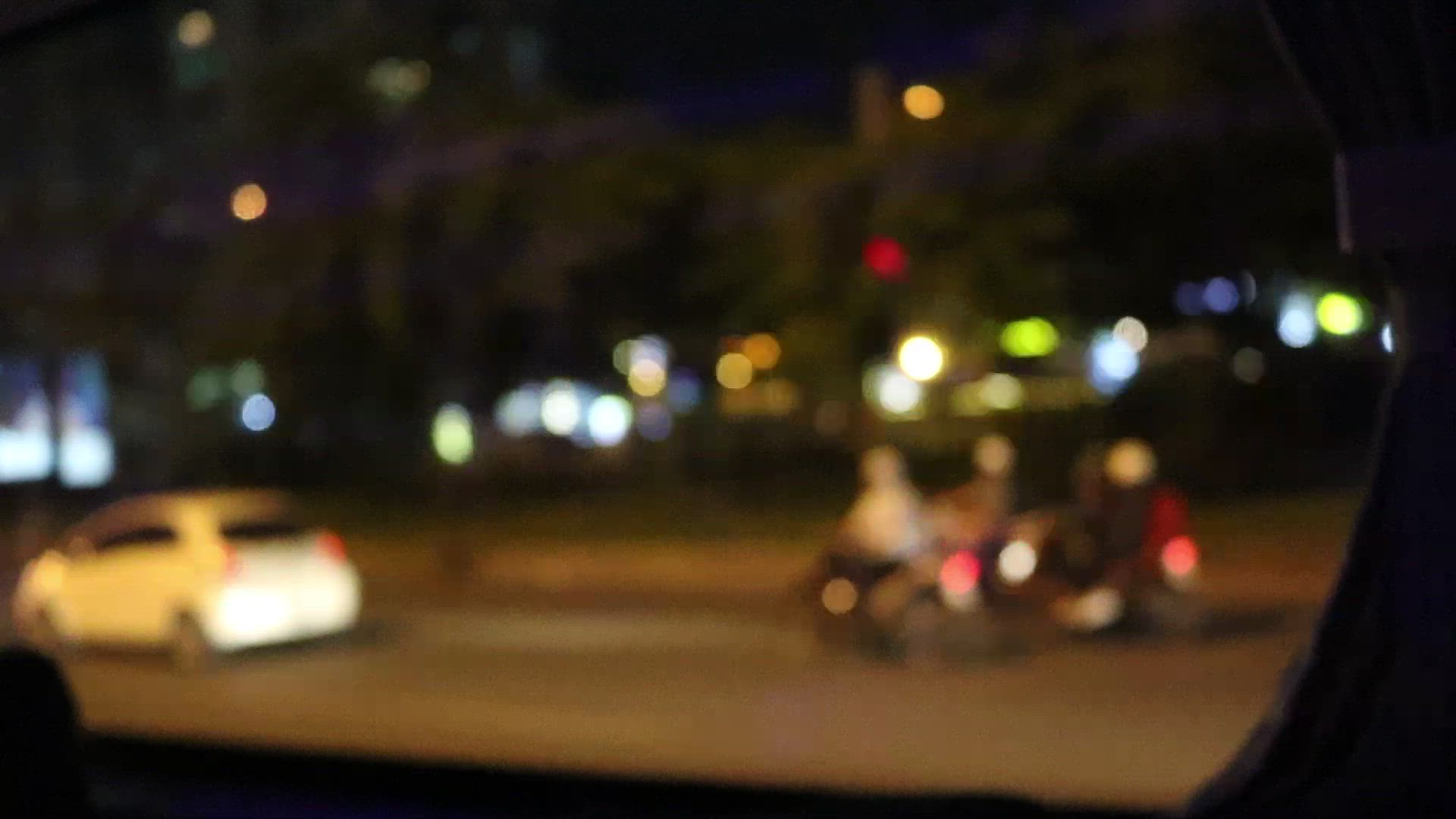This is a very blurry image taken at night through a car window, capturing a moving street scene. The photo features a white car with its red brake lights illuminated, traveling ahead on the right side of the road. Behind the car, there are two to three motorcycles, distinguished by their glowing red taillights and the white helmets of the riders, though all the details are out of focus. The window's interior trim appears gray, and outside, the road and curb are visible but blurry, with hints of white stripes and an orange curb. The background displays a series of multicolored city lights in shades of red, blue, white, yellow, green, and orange, accompanied by faint shapes of buildings and trees. The predominant color is a dark night sky, adding to the overall obscurity of the image.